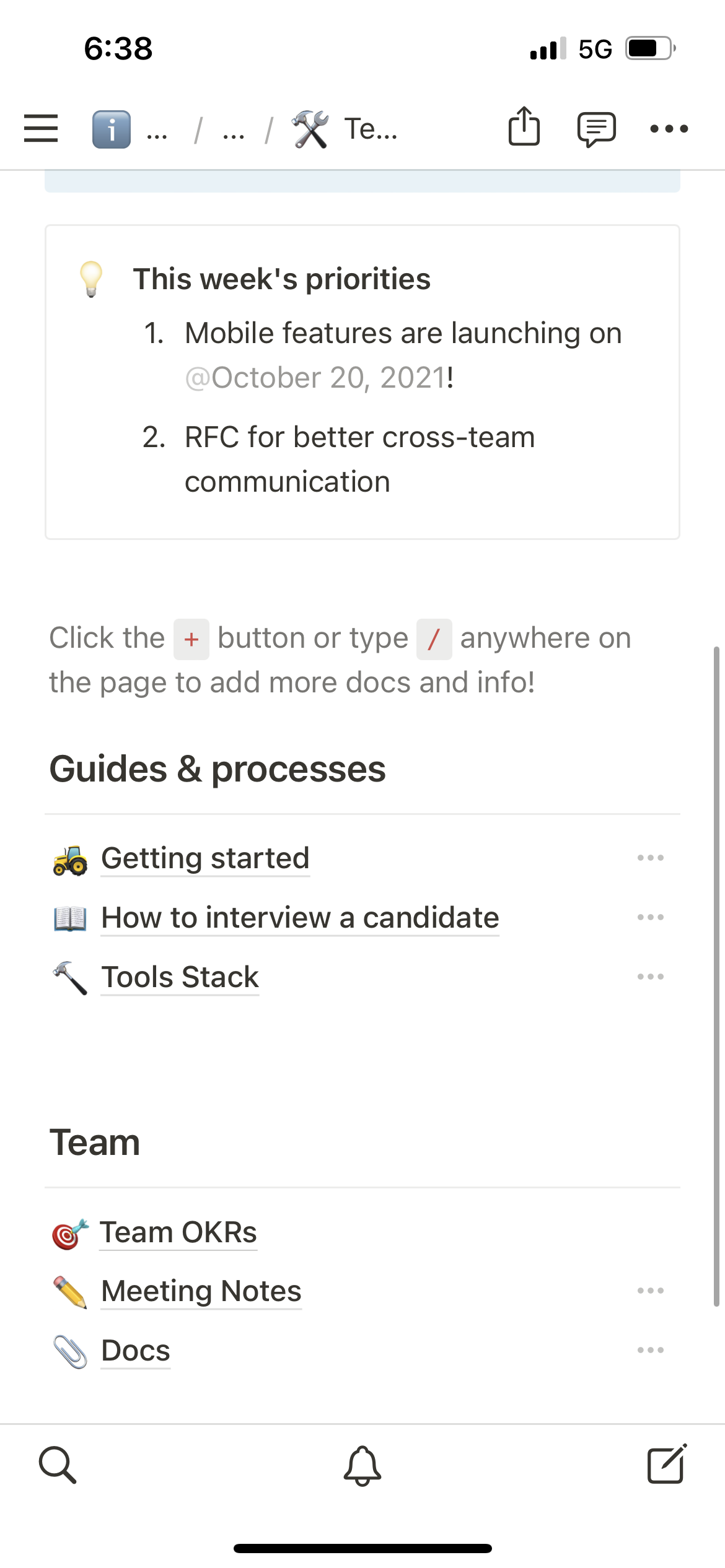This screenshot depicts the interface of an application, likely with automation features, in a portrait orientation. 

At the top of the screen, a white bar displays critical system information. On the left, the time reads "6:38," followed by a connection status showing 3 out of 4 bars, and a 5G icon. A horizontal battery icon indicates approximately 70% charge. 

Below this information bar, the interface includes a navigation menu with various icons: a hamburger menu for navigation, an information icon, slashes, a settings or tools icon, an upload button, a chat button, and an options menu symbolized by three dots.

The primary body of the screenshot features a white background, where a light bulb icon on the left highlights a section titled “This Week's Priorities.” It lists:
1. Mobile features launching on October 20, 2021.
2. RFC for better cross-team communication.

A prompt beneath this section advises users to "click the plus button or type backslash anywhere on the page to add more docs and info."

Subsequently, the content is divided into sections with headers. The “Guides and Processes” section includes categories such as:
- Getting Started
- How to Interview a Candidate
- Tool Stack

Each category is accompanied by relevant icons.

The “Team” section lists:
- Team OKRs
- Meeting Notes
- Docs

Each entry is also paired with corresponding icons.

At the bottom of the screenshot, three icons are visible: a magnifying glass for search, a notification bell, and a post icon for sharing updates or creating new entries.